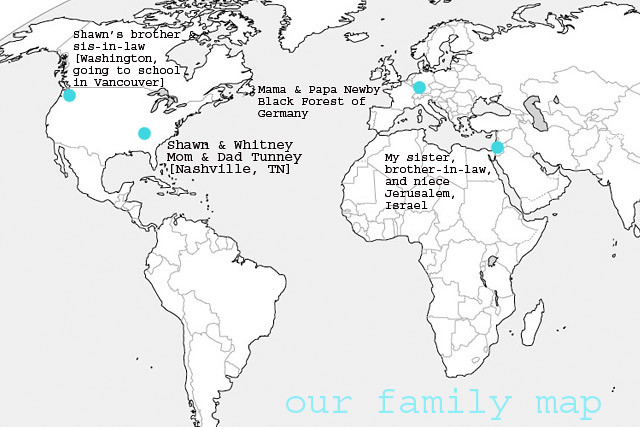The image is an outlined map displaying parts of North America, South America, Europe, Asia, and Africa with country borders in gray, while the landmasses are shown in white and the seas in gray. Titled "our family map" in a bright turquoise Courier font located in the lower right corner, the map includes several teal dots marking specific locations significant to the family. In North America, one dot near Washington represents Sean's brother and sister-in-law, who are going to school in Vancouver, while another dot in Nashville, Tennessee, identifies Sean and Whitney (mom and dad) Tunny. Across the Atlantic in Europe, a dot located in the Black Forest of Germany marks Mama and Papa Newby. Further east, a dot in Jerusalem, Israel, points to the residence of the speaker's sister, brother-in-law, and niece.